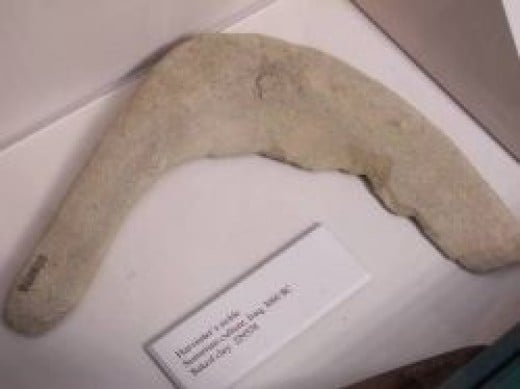The image depicts an ancient artifact shaped somewhat like a boomerang or sickle. It is positioned on a white backdrop, possibly a display box used in museums or for preservation purposes. The artifact, of a fossilized bone or baked clay color, appears old and slightly jagged at one end, suggesting it has deteriorated over time. There is an etching or a brand mark on the top left side of the object, which is hard to decipher from the image. Additionally, the artifact has a smaller rectangular note card placed above it on the white backdrop, raised slightly to provide a description. The note card, printed in small black font, identifies the artifact as a "Harvester's Sickle" from the Sumerian culture, dated around 3000 BC, and specifies its material as baked clay, marked with the number 229578. The overall presentation and descriptive elements indicate that this piece is a preserved relic likely displayed in a museum setting.